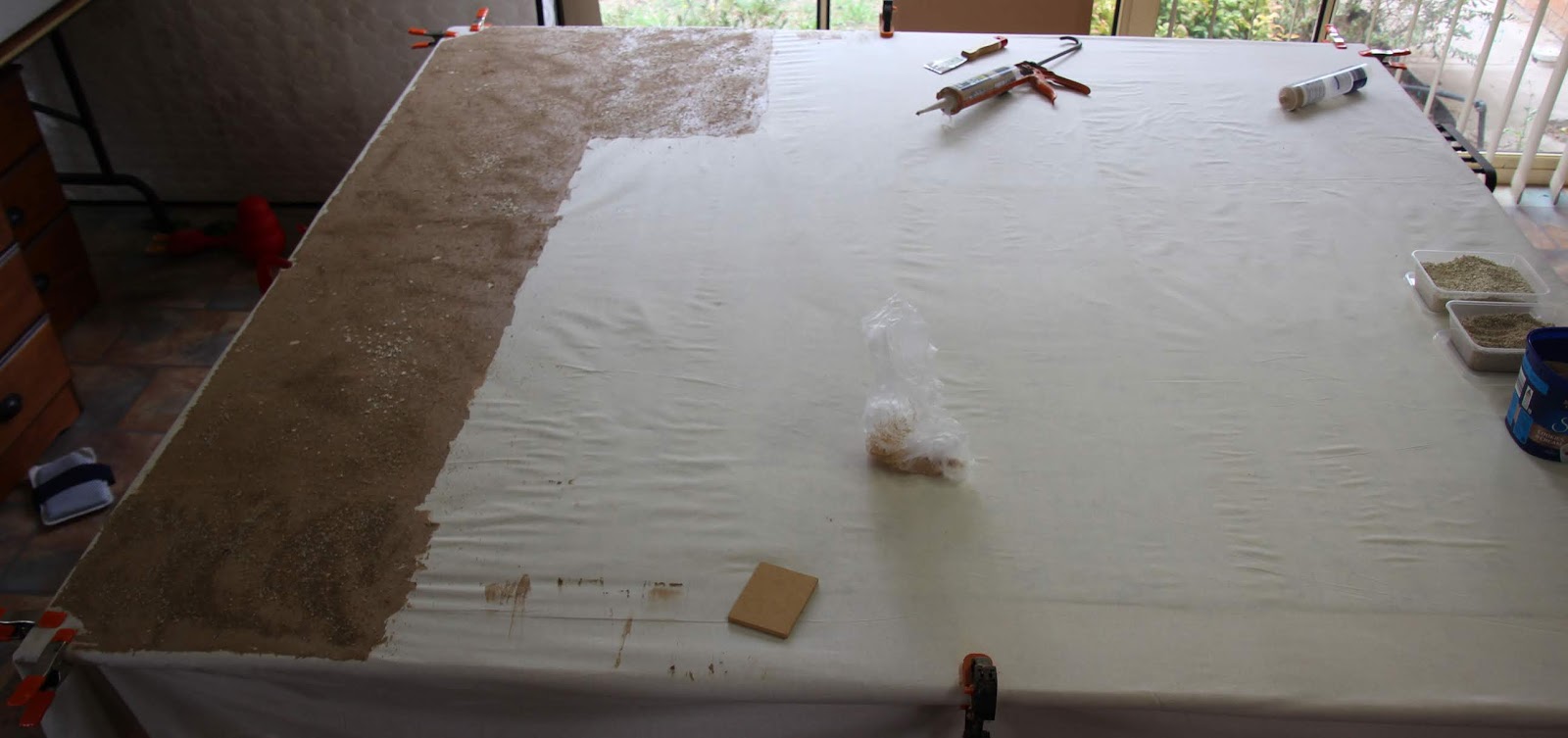In the photograph, a worktable is prominently featured, covered partially by a white sheet. On the left side of the sheet, there is a rectangular strip that has been painted a brownish color, and another section is in the process of being painted similarly. The tabletop hosts various tools, including a caulking gun and a scraping tool, indicative of construction or home improvement activities. Toward the bottom end of the table, there are two containers and a can, possibly holding paint or other materials. Clamps are visible at multiple points: securing the sheet to the table on the left and right edges, as well as at the corners near the top of the photograph. The surrounding environment includes glimpses of the floor and some furniture on the left, and structural elements like bars or framing on the right, suggesting that the work might be part of a home renovation project.